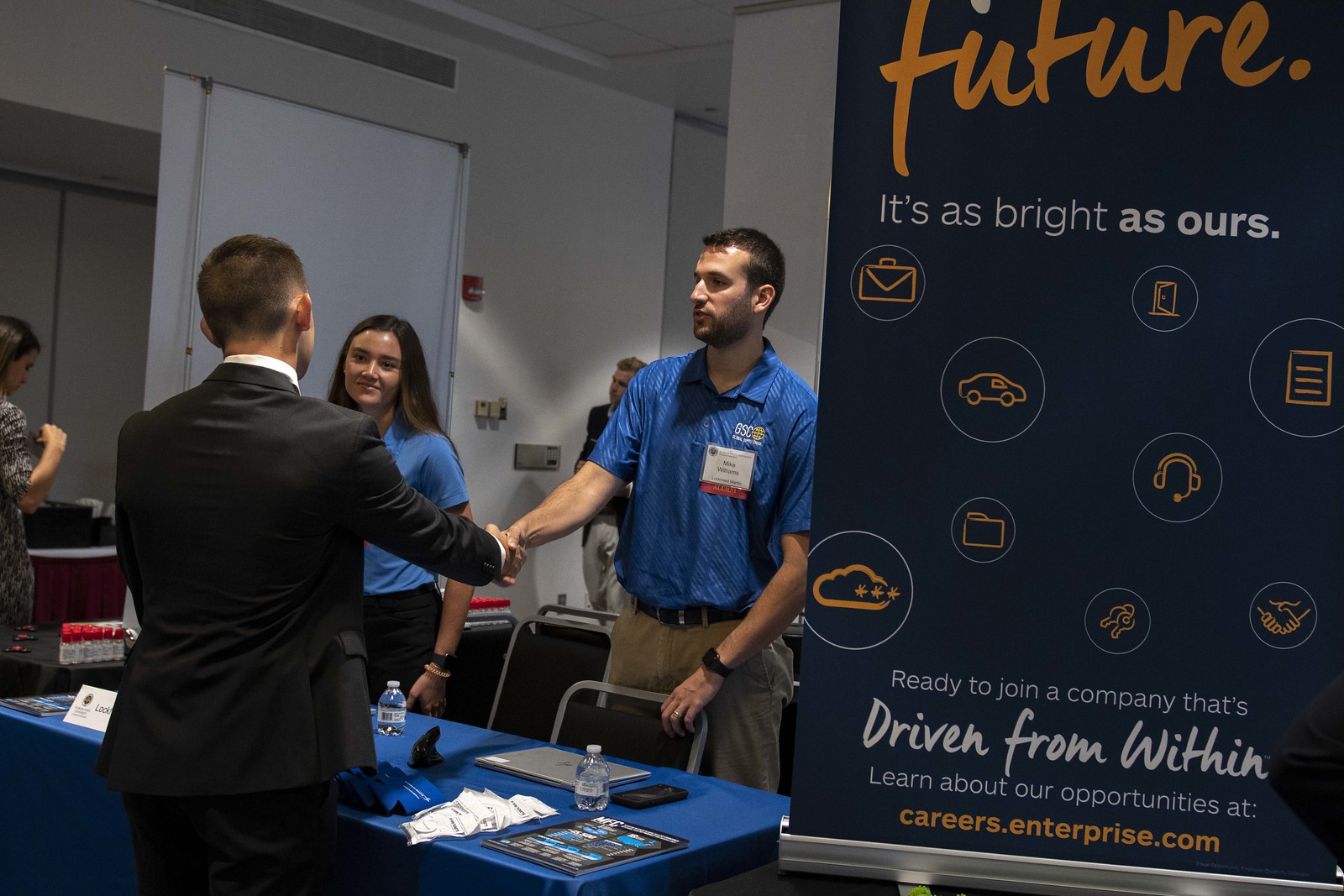This indoor photograph, taken at what appears to be a trade event or conference, captures a busy recruitment table for careers.enterprise.com. Central to the image are two representatives, a man and a woman, both dressed in blue shirts and work pants. The male representative, identifiable by his short brown hair and name tag that reads "Mike Williams" with "GSC" on his shirt, is warmly shaking hands with a potential candidate, who is dressed in an all-black suit with a white undershirt. The female representative with straight dark brown hair stands beside him, ready to engage with the attendees. 

The table, draped in a bright blue tablecloth, displays various branded merchandise, including can koozies, water bottles, a laptop, and a cell phone, all available as giveaways. In the background, a partially visible sign reads, "Future as bright as ours" and encourages attendees to explore opportunities at careers.enterprise.com. The scene is set within a room with white walls, and a few other people are faintly discernible in the background, contributing to the lively atmosphere of the event.